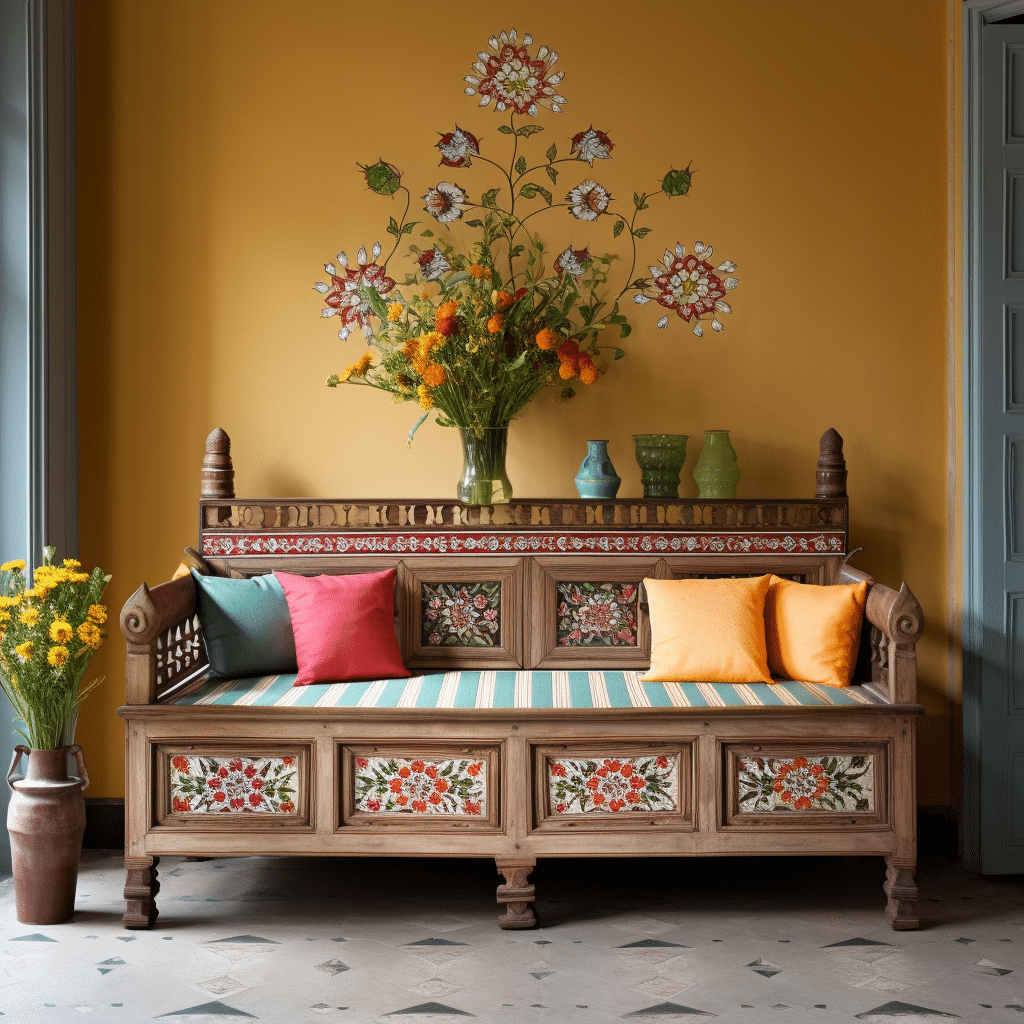This image showcases a meticulously curated sitting area, likely nestled within a garden room or a sitting room in a house. The vibrant setting features an elaborate two-seater sofa with a wooden frame, centrally positioned and facing the viewer. The sofa's wooden arms, feet, and back are intricately carved, and its frame is adorned with rectangular panels painted white, featuring red petaled flowers with green leaves. The seat cushion is patterned with light blue and white horizontal stripes, and it holds four square pillows — two teal and red pillows on the left, and two orange-yellow pillows on the right.

Dominating the background, an orange wall is adorned with painted flowers, featuring green stems, red flowers, and white petals, adding a cheerful and artistic touch. Above the sofa, a glass vase brims with a dense bouquet of flowers, showcasing an array of colors with orange, red, and yellow blooms and lush green stems. To the right of this vase, three smaller empty vases in varying shades of light blue, green, and olive are placed on a built-in shelf of the sofa.

The flooring in front of the sofa appears to be either a thin carpet or hardwood, setting a neutral base for the vibrant scene. On the floor, to the left of the sofa, there is a brown vase—possibly metal or ceramic—holding tall flowers with thick yellow petals and long green stems. This detailed composition, brimming with rich colors ranging from greens, reds, oranges, yellows, blues, whites, and browns, transforms the sitting area into a visually engaging and cozy space.